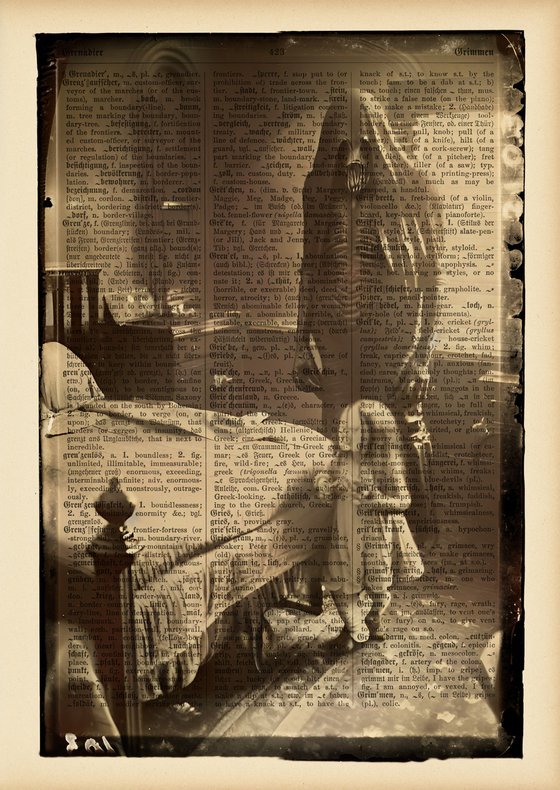The image presents a haunting scene, characterized by a tan background displaying an illegible article, likely in a foreign language. Overlapping this text is a double-exposure style black-and-white photo of a bedroom. Central elements include a wooden four-post bed on the left, a dresser in the corner, and a carpeted floor. A toddler girl with long hair and a knee-length dress is seen walking obliviously across the room, her face lacking discernible features. Looming menacingly behind her is a ghoul-like figure with a hood covering its skeletal, bony face, sharp teeth, and ribcage visible through tattered clothing, extending eerie, elongated fingers toward the child. The overall composition evokes an unsettling, spooky atmosphere.